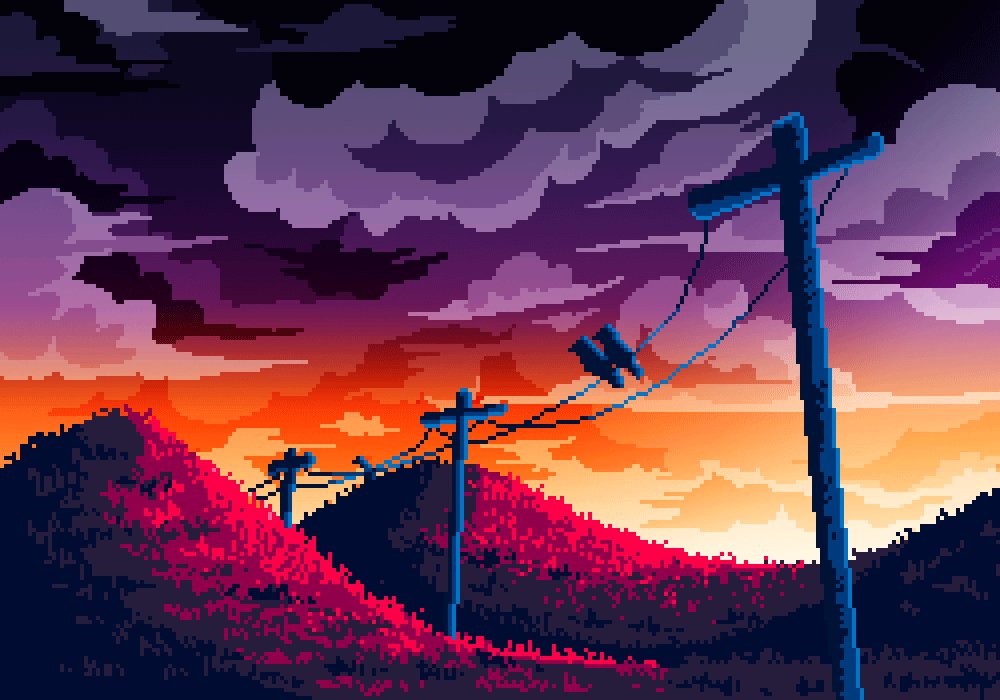The image is a horizontal, low-resolution landscape reminiscent of pixel art, likely created in MS Paint. The top half features a vibrant purple gradient sky dotted with grey clouds, transitioning into a warm orange and yellow horizon. Below, the landscape is composed of three hills: two fully visible on the left and one partially shown on the right. These hills are speckled with red, suggesting the warm glow of a sunset. Blue telephone poles span from the bottom left towards the upper right, with wires connecting them across the undulating terrain. This pixelated, yet colorful depiction captures the essence of a serene countryside at dusk.